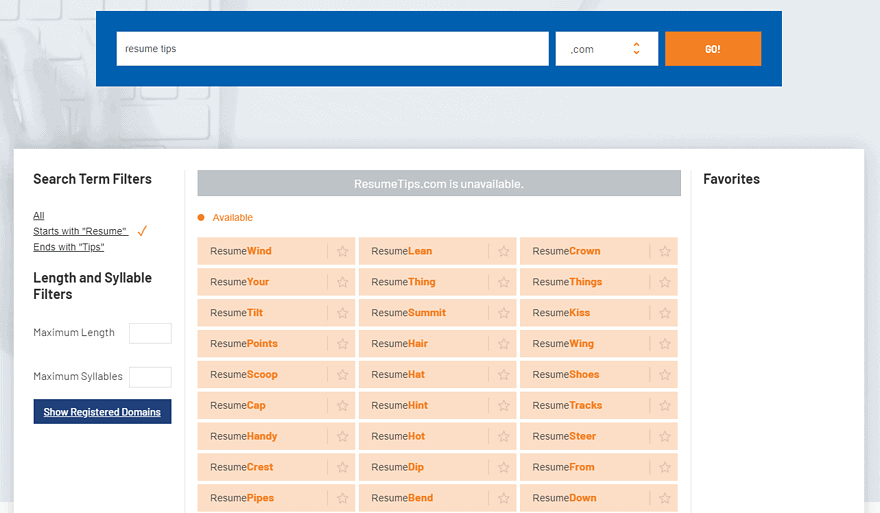A web page designed for job searching is prominently displayed. At the very top, there is a large blue rectangular banner with a search field in its center. In the search field, the phrase "resume tips" has been entered. Adjacent to the search box, on the right, is a drop-down menu set to ".com", allowing users to search various domains such as .com, .gov, and others for resume tips. To the right of the drop-down menu is an orange "Go" button to initiate the search.

Below this search area are the search results. To the left of the search results is a column labeled "Search Terms Filters," offering options to further refine the results. The first filter option is labeled "All Results." The second filter option, "Starts with a resume," is selected by default, indicated by a check mark. The third filter option is "Ends with tips (t-i-p-s)." Additional filters include syllable filters and options to set maximum length and minimum syllables.

Beneath these filters is a blue button labeled "Show Registered Domains." An indication is provided that the domain "resumetips.com" is unavailable.